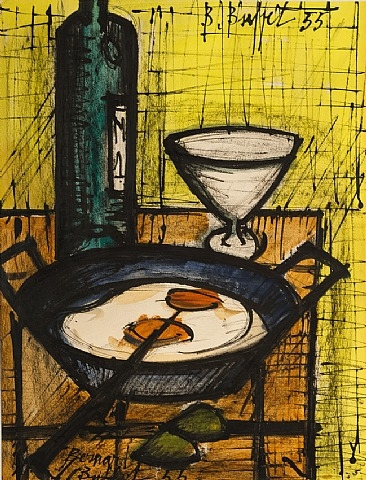This detailed painting portrays a kitchen scene set indoors. Dominating the composition is a brown table with a black border, contrasting against a vivid green backdrop. At the center of the table rests a black, cast-iron skillet bearing two perfectly cooked sunny-side-up eggs. Behind the skillet, a triangular-shaped wine glass appears, paired with a green bottle to its left. The bottle's label intriguingly suggests text with an "M" and possibly the number "4," and notably features the painter's name "B. BUFFET 55" at the top. The scene is framed by a wall awash in diverse colors, primarily yellow, marked with black scribbles and scratches, adding a dynamic texture. The overall aesthetic highlights the painter’s bold use of shading, color contrasts, and striking black outlines, creating a visually engaging and richly detailed artwork.